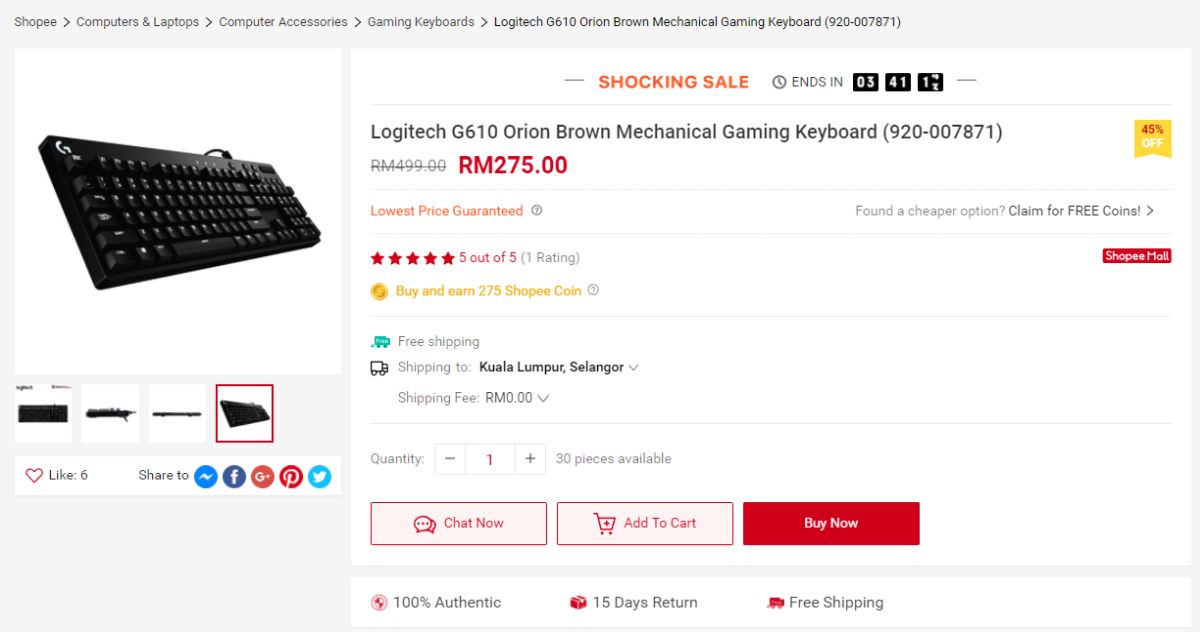The image is a screenshot of a web page featuring a Logitech G610 Orion Brown mechanical gaming keyboard. At the top of the web page is a navigation path showing the following categories: Shop > Computers & Laptops > Computer Accessories > Gaming Keyboards > Logitech G610 Orion Brown Mechanical Gaming Keyboard, along with an item number. The left-hand side of the screen displays an image of the keyboard itself, shown from above to highlight its deep keys, in black and white.

Below the image is an option to 'heart' the item, which indicates it has been liked six times. There are also social media share buttons for Pinterest, Twitter, Google+, Facebook, and Messenger. 

An orange banner announces a "Shocking Sale" that ends in three hours and 41 minutes. The keyboard is being sold at a 45% discount, bringing the price down to RM275.00, the lowest price guaranteed. It has a perfect five out of five stars rating and qualifies for free shipping, specifically to Kuala Lumpur and Selangor, with the shipping fee shown as zero.

At the bottom of the page, there are three prominent buttons: "Chat Now," "Buy Now," and "Add to Cart."